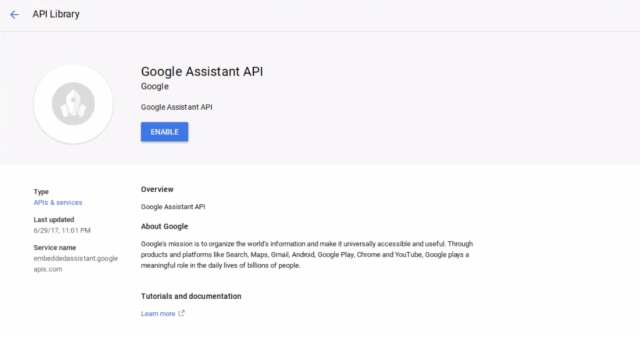In the image, the top section features a light gray rectangle with an arrow pointing left on the top-left corner, which is labeled "API Library." Beneath this, a horizontal gray line extends across the full width of the rectangle. Below the line, a white circle is centered with a gray circle inside it. Within the gray circle, a white spaceship-like icon is depicted. Just below this circular arrangement, the text reads "Google Assistant API" followed by a smaller "Google" underneath. Further down, there is a line of small, unreadable text. Directly under this text, a prominent blue rectangle displays the word "Enable."

The area beneath the blue rectangle is white, containing text that's challenging to decipher due to its size. On the left, there is black text followed by blue text beneath it, and further black text under that. To the right, more black text is present, leading into a paragraph written in black. Following the paragraph, there are additional lines of small black text, interspersed with portions of blue text.

Upper-right of the detailed section, there is an icon resembling a partial circle with an arrow pointing upwards and to the right. This part of the image includes partially readable categories, with "Type" at the top and "Overview" next to it on the right. Below "Overview," there is additional blue text, but the precise wording is illegible. Underneath the section labeled "Overview," the text "Google Assistant" is partially visible, though the rest remains unreadable. The image features numerous small text elements that are too tiny to distinguish clearly.